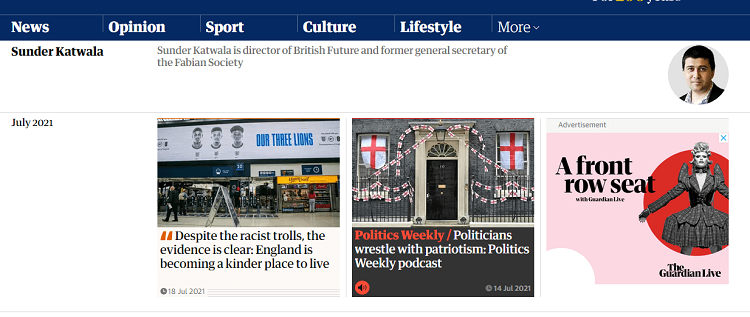The image showcases a news webpage with a dominant blue header at the top featuring six clickable links: News, Opinion, Sport, Culture, Lifestyle, and a "More" option accompanied by a drop-down arrow. Just below the header, there is a horizontal white box containing the bold black text "Sunder Katwala." A brief biographical note states that Sunder Katwala is the Director of British Future and a former General Secretary of the Fabian Society. Adjacent to this text, there is a circular photograph of Sunder Katwala, depicting a darker-skinned individual with short black hair, a clean-shaven face, dressed in a black and white suit. Below his image, "July 2021" is noted.

Further down, three distinct news links are presented. The first link, on the left, features an image of a storefront with blue and yellow hues and a tiled floor. The caption reads: "Despite the racist trolls, the evidence is clear: England is becoming a top gander place to live." The central link presents an image of a red cloth below a white flag, with the description: "Politics Weekly: Politicians wrestle with patriotism - Politics Weekly Podcast." The background comprises a significant building adorned with flags. On the right, there is a pink backdrop with a red circle, featuring what appears to be Lady Gaga in the center, possibly next to a white, unusually shaped statue. The caption includes: "A front row seat with [unreadable name]" followed by "The Guardian Live" on the bottom right-hand corner.